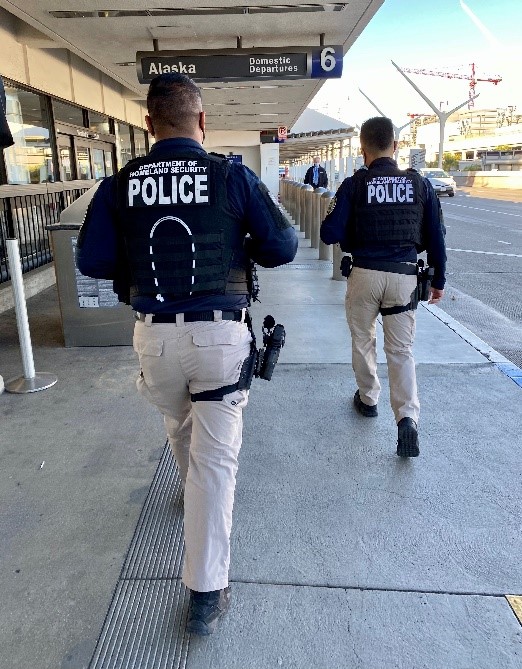The photograph, taken outdoors during the daytime, captures two police officers walking away from the camera along a sidewalk adjacent to a small roadway. The officers, wearing light khaki pants with gun holsters strapped to their thighs, are dressed in dark blue long-sleeve shirts with black bulletproof vests that read "Department of Homeland Security Police" in white print on the back. Their black shoes contrast with their pants. To the left of the officers is a large building with windows, and they are walking under an overhang. A sign above them reads "Alaska Domestic Departures Terminal 6." The scene suggests an airport setting with visible airline signs. A car travels in their direction on the road, which features white lines, while another officer dressed in a dark jacket and blue shirt approaches from the background. Further along the sidewalk, pylons separate it from the road, and a parking sign is visible above them. Additionally, a crane is noticeable above another building to the right of the image.